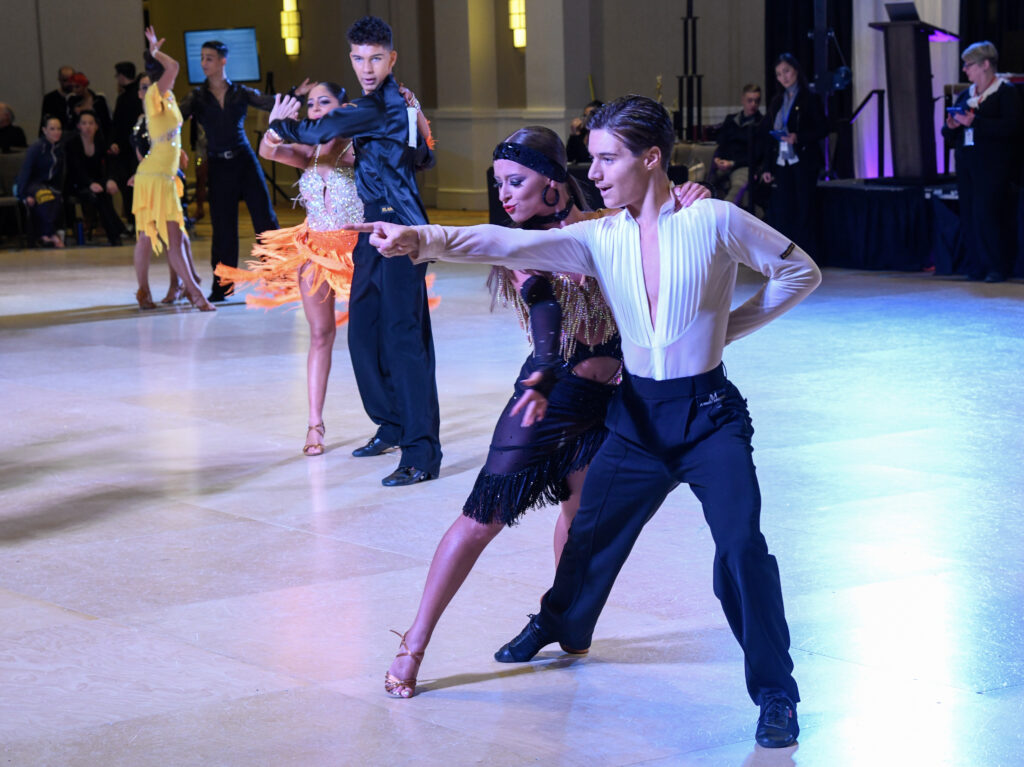This vibrant indoor scene captures a lively ballroom dance competition, set within a brightly lit arena. In the foreground on the right side, a Caucasian couple commands attention with their poised stance. The gentleman wears black trousers and a white collared shirt with an open neck, pointing left with his right arm while holding his partner's hand behind his back. The elegant woman by his side has long blonde hair, adorned in a short black Latin-style dress with fringes, paired with gold high-heeled sandals. She gazes left, aligning her stance perfectly with her partner's direction.

At the center of the polished white tile dance floor with subtle blue lighting, another dynamic couple radiates energy. The young man, dressed in black trousers and a striking blue long-sleeve shirt, looks directly into the camera. His arm extended, he holds the hand of his partner, a young Caucasian woman with dark hair pulled back. She dazzles in a white sequined bodice with a vibrant orange feathered skirt that flares elegantly, indicating a recent twirl. She too wears gold high-heeled open-toed sandals.

In the distant background, a third couple performs near the far end of the floor. The gentleman sports a black long-sleeve shirt and black pants, while his partner dons a bright yellow Latin dress with long fringe. Her arms stretch gracefully above her head as they move in unison.

Surrounding the dance floor, spectators sit against tall beige walls, captivated by the performances. By the stage, located at the top right corner of the photograph, a few individuals stand, possibly awaiting their turn or judging the event. A table in the middle holds trophies, promising rewards for the night's top performers. The entire scene is rich with the vibrant costumes and coordinated movements characteristic of an exhilarating ballroom dance competition.